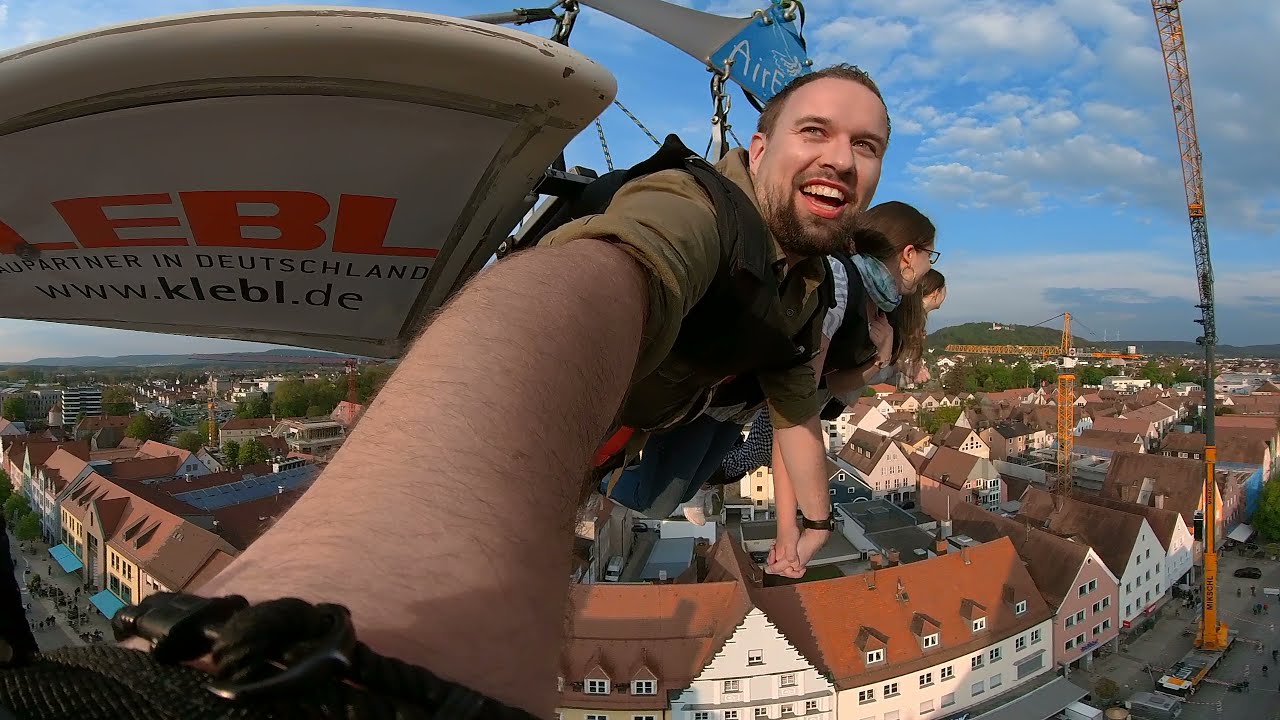The image captures an exhilarating moment of three people, a man and two women, on an amusement ride resembling a parasailing or zipline experience. The man, who has short brown hair, a short brown beard and mustache, and is wearing a dark green shirt, is holding a camera with his arm extended, creating a vibrant selfie. They're all securely strapped in black harnesses to a large, industrial, yellow and black crane arm that extends into the sky. The scene is set high above a residential area filled with white buildings adorned with red and brown tiled roofs, showcasing triangular pointed designs. In the background, a picturesque mountain range with lush green trees punctuates the horizon under a mostly blue sky with scattered white and gray clouds. Part of the ride's white wing, featuring orange and blue text and a website address, is visible at the top left corner of the image, adding to the sense of adventure and height.